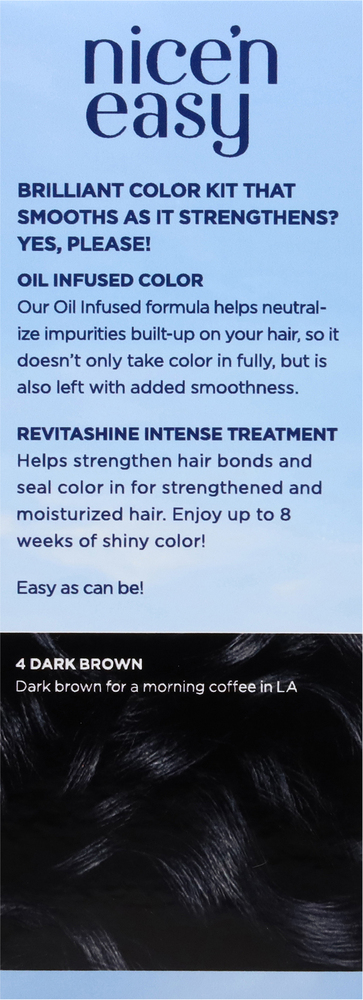This image features a detailed advertisement for a hair color treatment product. The background is a light blue color, and at the top, it prominently displays the phrase "Nice 'n Easy." Below this, it boasts a "Brilliant Color Kit That Smooths as It Strengthens, Yes Please!" and emphasizes its "Oil Infused Color." The ad describes how their oil-infused formula helps neutralize impurities built up on your hair, ensuring that not only is the color fully absorbed, but your hair is also left with added smoothness. Next, it highlights the benefits of the "RevitaShine Intense Treatment," which aids in strengthening hair bonds and sealing in color, resulting in moisturized hair. The treatment promises up to 8 weeks of shiny, vibrant color, making the coloring process "Easy as Can Be." At the bottom of the advertisement, there is a close-up image of dark brown hair with the text "For Dark Brown," followed by "Dark Brown for a Morning Coffee in L.A." The hair depicted is an extremely dark brown shade, almost approaching black.